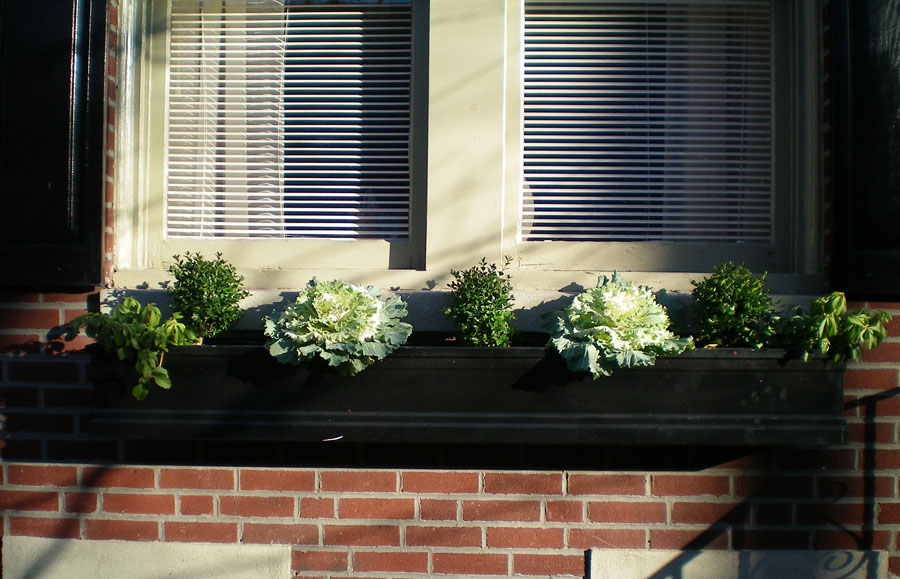The image features the exterior of a well-maintained red brick house with a double window that has white trim and a thick wood frame. The windows are adorned with black shutters on each side and are fitted with white blinds and floor-to-ceiling drapes visible from the inside. Beneath the window sits a long, black planter box, hanging securely and filled with what appears to be various types of cabbages, lettuces, and possibly other herbs or vegetables, suggesting an ornamental or decorative purpose rather than for consumption. The bricks below the window display faint white images or markings, and the shadows cast by some sort of railing or wrought-iron handrail are visible. Additionally, on the lower portion of the brick wall, there are two gray concrete-like squares.